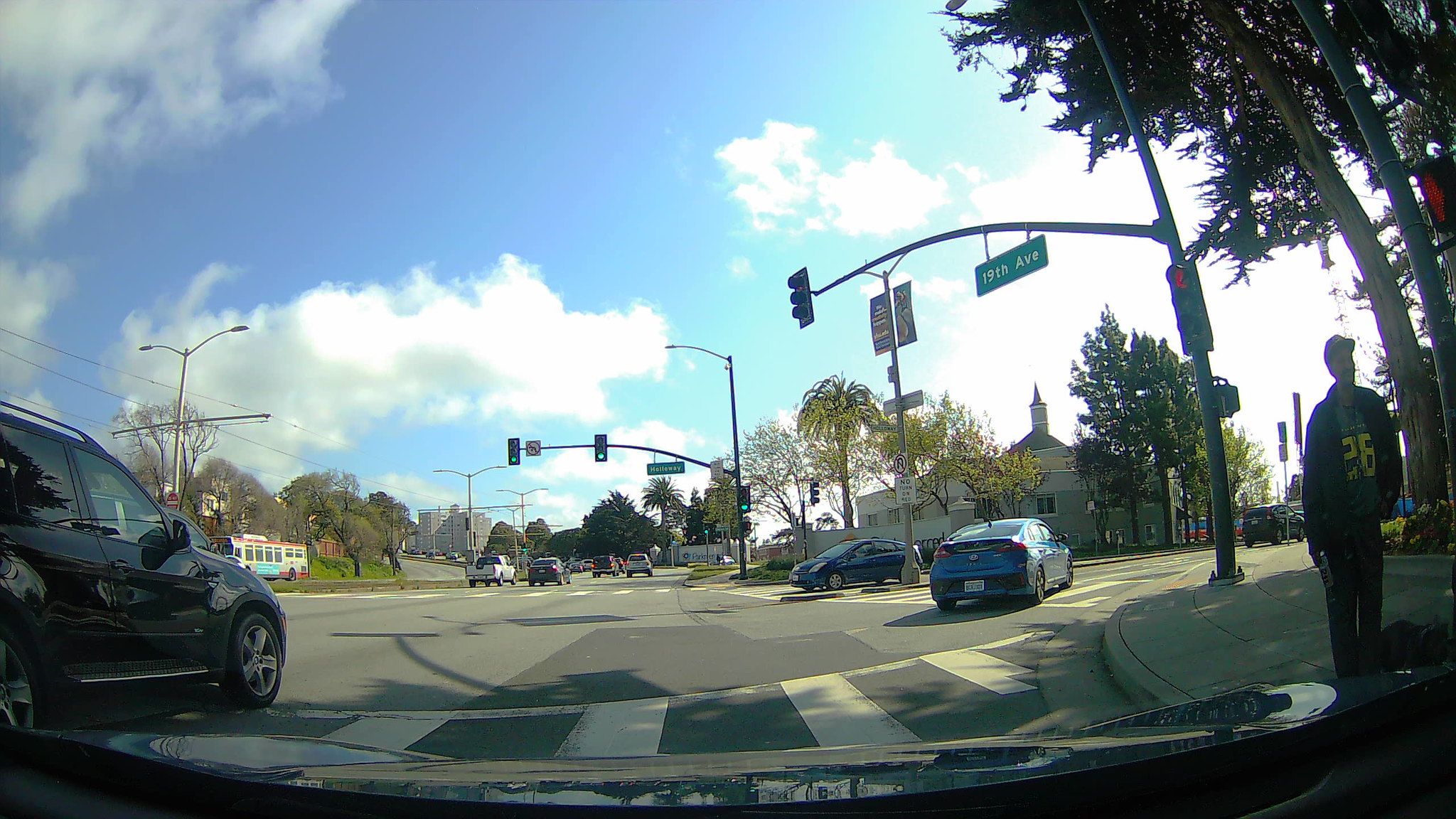The image captures a busy street corner bustling with activity. Prominently featured are two sets of traffic lights: one situated on the right-hand side of the image, affixed to a light pole along with a green street sign that reads "19th Avenue," and another set positioned in the background, centrally located. The scene includes approximately six to seven vehicles in various stages of transit—some maneuver through the intersections, others turn, a few have already passed the background traffic lights, and several wait for their cue to move. On the left-hand side is a bus, further contributing to the urban atmosphere. The sky above is a serene blue dotted with a few clouds, adding a touch of calm to the otherwise dynamic street scene. In the bottom right-hand corner, a gentleman is spotted walking along the sidewalk, enhancing the everyday slice-of-life feel of the image.